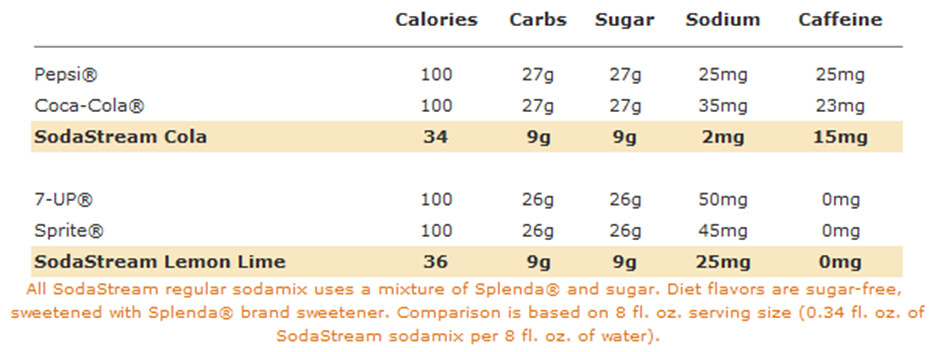This image depicts a detailed spreadsheet that compares various soda products based on their nutritional content. The rows are labeled with different soda brands: Pepsi, Coca-Cola, SodaStream Cola (highlighted in a brownish-yellow color), 7-Up, and Sprite. Additionally, SodaStream Lemon Lime is highlighted in a yellowish color. The table includes columns for calories, carbs, sugar, sodium, and caffeine.

The purpose of this comparison is to demonstrate the health benefits of SodaStream products relative to other popular sodas. According to the table, all SodaStream regular soda mixes use a combination of Splenda and sugar, while their diet flavors are completely sugar-free, sweetened solely with Splenda brand sweetener. The comparison is standardized to an 8 fluid ounce serving size, which equates to 0.34 fluid ounces of SodaStream soda mix per 8 fluid ounces of water. A note at the bottom of the spreadsheet, written in an orangish color, provides this specific information about the serving size and sweetening agents used in SodaStream products.